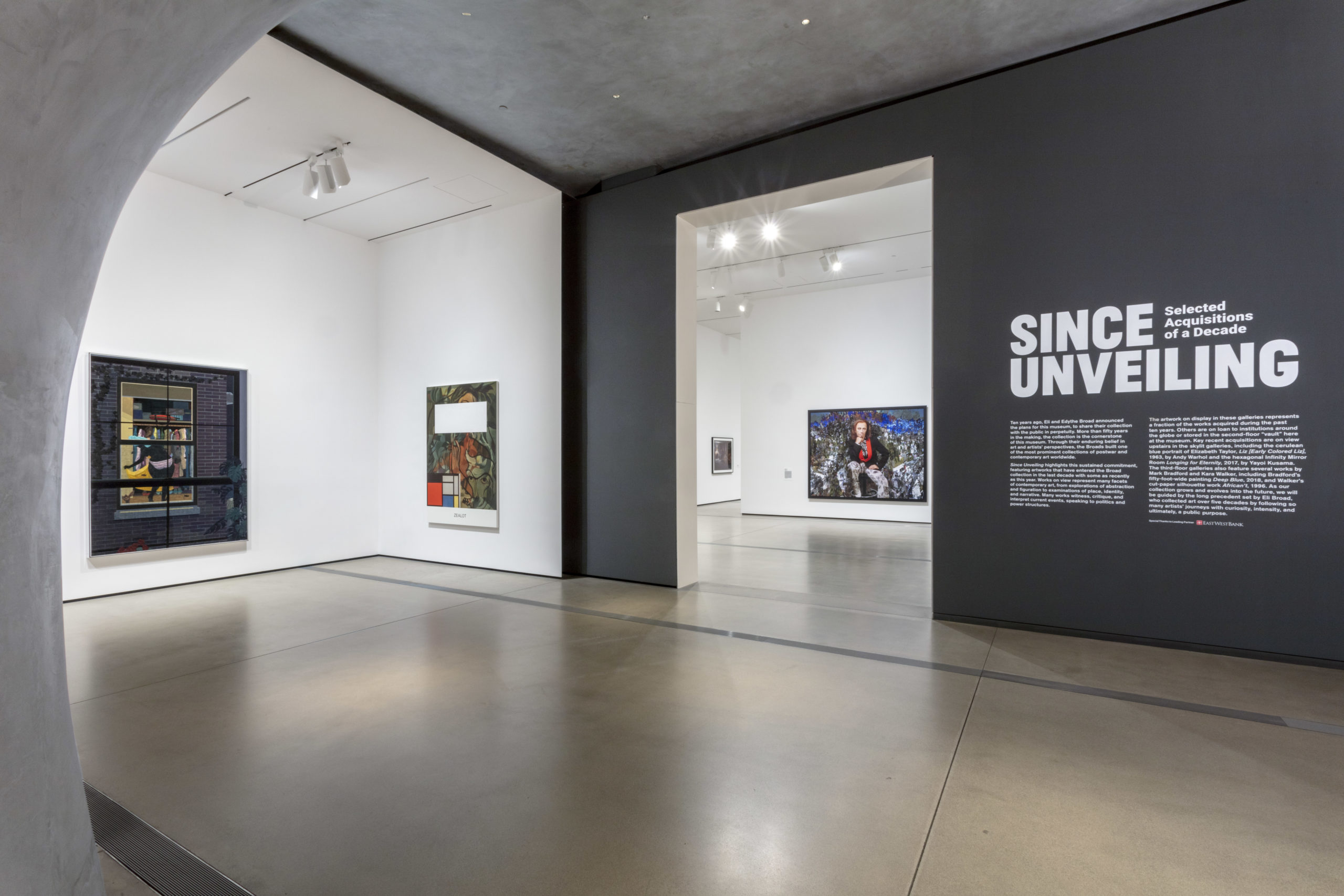The image displays a spacious, contemporary art gallery with a polished concrete floor. The left side features a boxed, white-walled room adorned with abstract paintings that exhibit vibrant colors. The white ceiling in this section is fitted with three overhead lights that illuminate the space. Among the artworks on the white wall, one particularly dark piece resembles a view through a window at someone sitting by a bookcase. Adjacent to it, another art piece remains indistinct. On the right side, a large dark gray wall stands, inscribed in prominent white lettering with the words "Since Unveiling: Selected Acquisitions of a Decade," followed by smaller text detailing the gallery's acquisitions, though the script is too small to decipher. This gray wall also features an open frame doorway that leads to another section of the building, where more art pieces hang on pristine white walls. The ceiling above the gray wall appears to be gray cement, contrasting with the various textures and surfaces throughout this multifaceted gallery space.